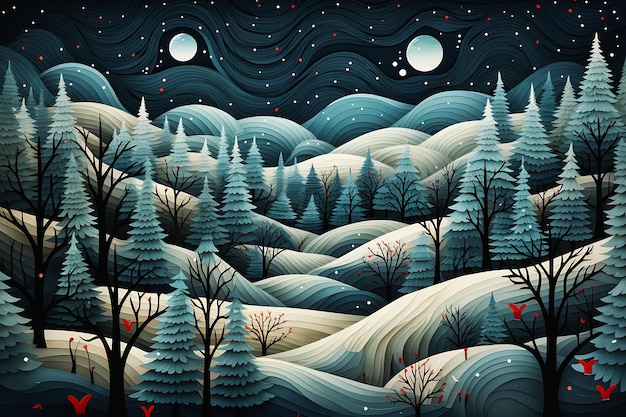This horizontal rectangular image is an artist's rendition of a magical land that evokes a sense of whimsy and wonder, reminiscent of a holiday greeting card. The sky, an enchanting black backdrop filled with an abundance of white and occasional blue, red, and yellow stars, is dominated by two moons; the larger one sits on the right while the smaller one is positioned on the left. Wave-like patterns infuse the sky with dynamic movement, enhancing its surreal quality.

The landscape beneath features a series of undulating green and white lumps that resemble corduroy fabric swells and elongated hills, respectively. Green mounds are more rounded, and the white ones stretch out gracefully. Stretching from the horizon down to the foreground, these lumps form a tiered terrain that creates a captivating depth in the image.

Interspersed throughout the scene are various trees. The ones on the left and right sides are particularly dense, comprising both symmetrical, light-blue spruce-like trees and bare-branched deciduous trees. These trees add a festive, almost wintry vibe, reminiscent of a Christmas scene. Furthermore, scattered across the landscape are intriguing red marks, potentially representing small birds or festive ornaments, adding a pop of color to this serene and mystical landscape.